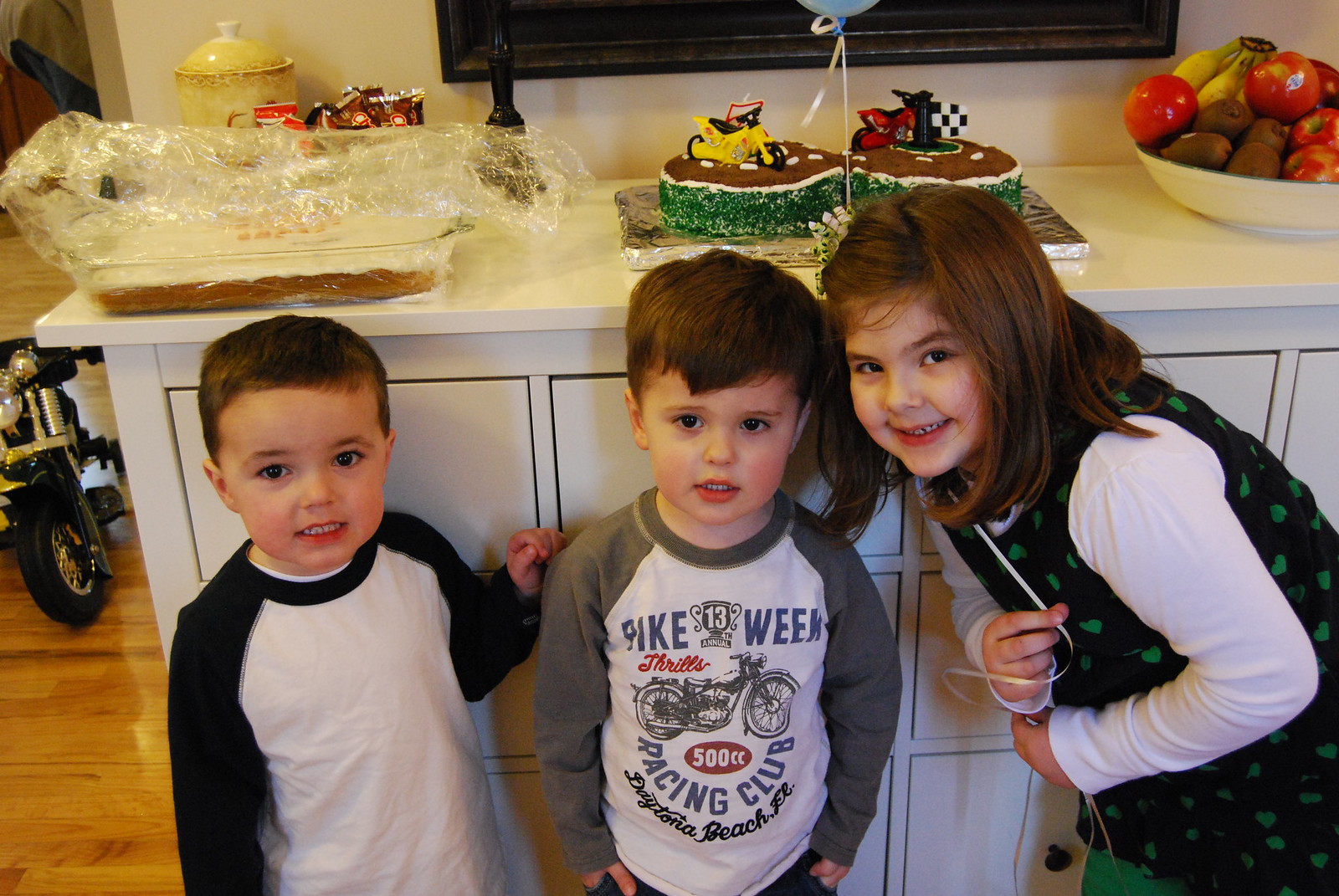This vibrant photograph features three children standing in front of a white counter, likely in a bakery or café. The colorful scene is accentuated by the various fruits and cakes neatly arranged on the counter. The children, dressed in casual, colorful outfits, are smiling and facing the camera. On the left, a boy with brown hair wears a black and white t-shirt, standing in front of a white cabinet. In the center, a dark-haired boy sports a gray and white t-shirt emblazoned with the words "racing club" and a motorcycle graphic. On the right, a girl wearing a black and green outfit over a white long-sleeve shirt is smiling and leaning slightly over the boy in the middle, holding a white ribbon attached to a blue balloon floating above.

The counter behind them boasts an assortment of items: a bowl filled with apples, kiwis, and bananas; a birthday cake designed as a racetrack with red and yellow motorcycles on a brown track; another dessert covered with saran wrap in a glass cake pan; a small bowl of chocolates; and a yellow vase. Below, the shiny yellow wooden floor adds to the cheerful ambiance, with a small toy resembling a motorcycle visible on the left side.